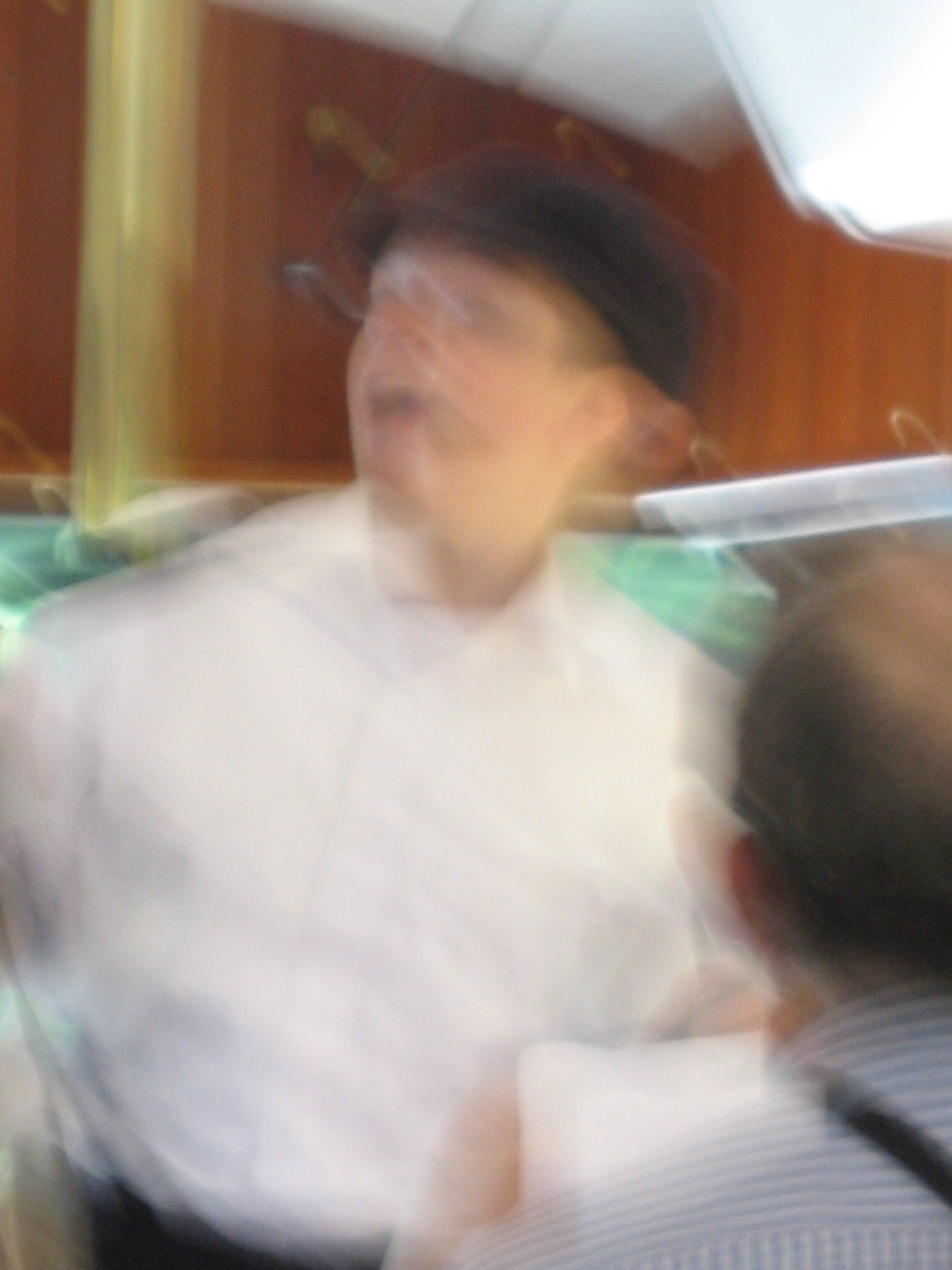In this blurry photograph, a person with a Caucasian skin tone is captured from the waist up. The individual is wearing a black hat and a white button-down shirt. Black pants are also visible. In their right hand, they appear to be holding something white. The background of the image features brown walls and what seems to be a white ceiling. There is white trim visible on both the right-hand side of the frame and behind both shoulders. Behind the person’s shoulders, there are noticeable green triangular shapes, although their exact nature is unclear due to the blur.